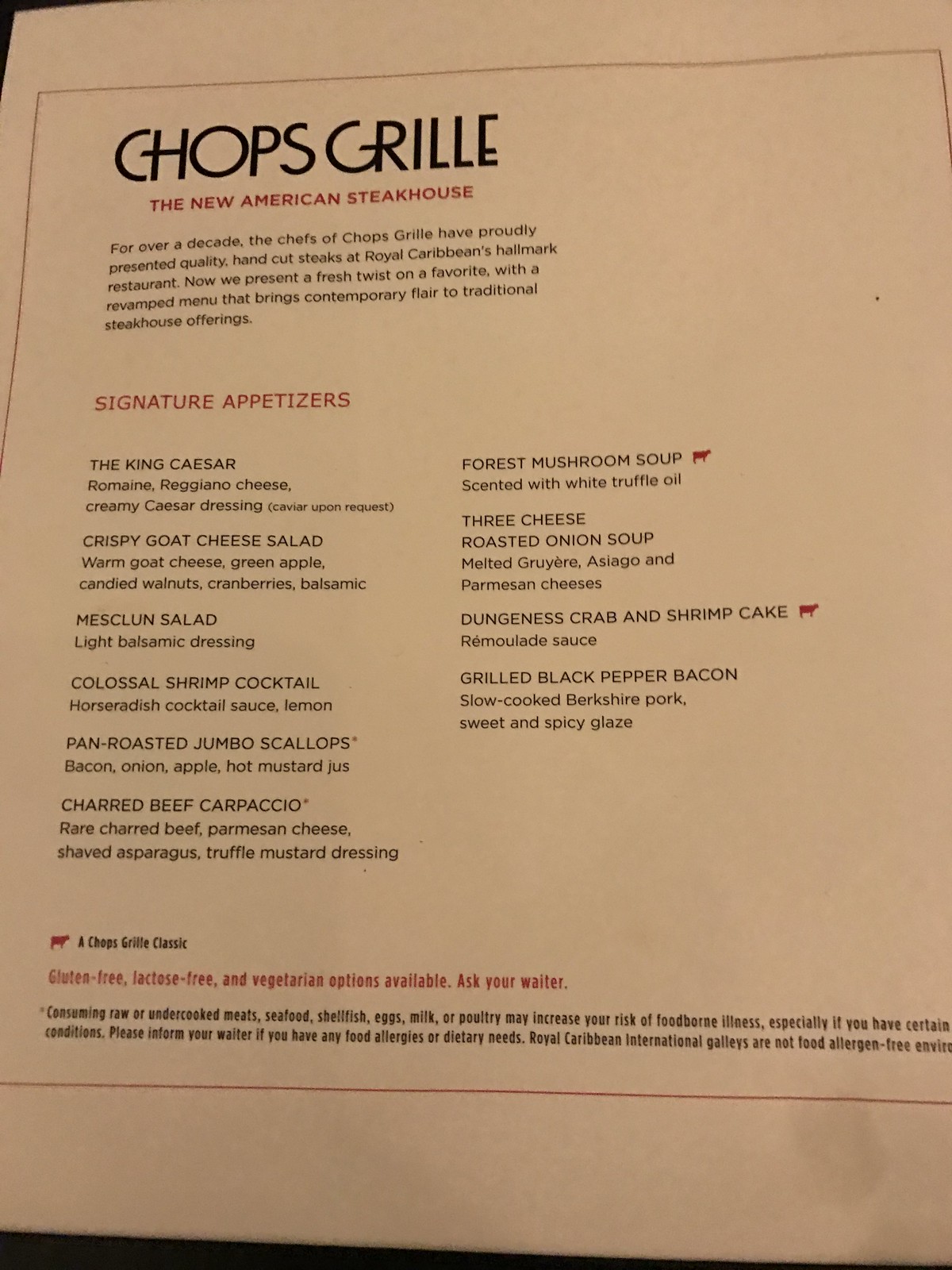**Chops Grille New American Steakhouse Menu**

This vibrant color photograph showcases the elegant menu of Chops Grille, The New American Steakhouse. At the top, the restaurant name "Chops Grille" is prominently displayed, followed by the tagline, "The New American Steakhouse." The introduction reads: "For over a decade, the chefs of Chops Grille have proudly presented quality hand-cut steaks at Royal Caribbean's hallmark restaurant. Now, we present a fresh twist on a favorite with a revamped menu that brings contemporary flair to traditional steakhouse offerings."

**Signature Appetizers:**

- **The King Caesar:** Romaine, Reggiano cheese, creamy Caesar dressing, caviar upon request.
- **Crispy Goat Cheese Salad:** Warm goat cheese, green apple, candied walnuts, cranberries, balsamic, mesclun salad, light balsamic dressing.
- **Colossal Shrimp Cocktail:** Horseradish cocktail sauce, lemon.
- **Pan-Roasted Jumbo Scallops:** Bacon, onion, apple, hot mustard jus.
- **Charred Beef Carpaccio:** Rare charred beef, parmesan cheese, shaved asparagus, truffle mustard dressing.
- **Forest Mushroom Soup:** Scented with white truffle oil (denoted with a red cow icon).
- **Three Cheese Roasted Onion Soup:** Melted Gruyere, Asiago, and Parmesan cheeses.
- **Dungeness Crab and Shrimp Cake:** Remoulade sauce (denoted with a red cow icon).
- **Grilled Black Pepper Bacon:** Slow-cooked Berkshire pork, sweet and spicy glaze.

At the bottom of the menu, a description about the red cow icon notes: "This denotes a Chops Grille classic." It also mentions the availability of gluten-free, lactose-free, and vegetarian options, advising guests to ask their waiter. The important health advisory states, "Consuming raw or undercooked meats, seafood, shellfish, eggs, milk, or poultry may increase your risk of foodborne illness, especially if you have certain..." though the line is cut off.

The final note reads: "Please inform your waiter if you have any food allergies or dietary needs. Royal Caribbean International galleys are not food allergen-free environments."